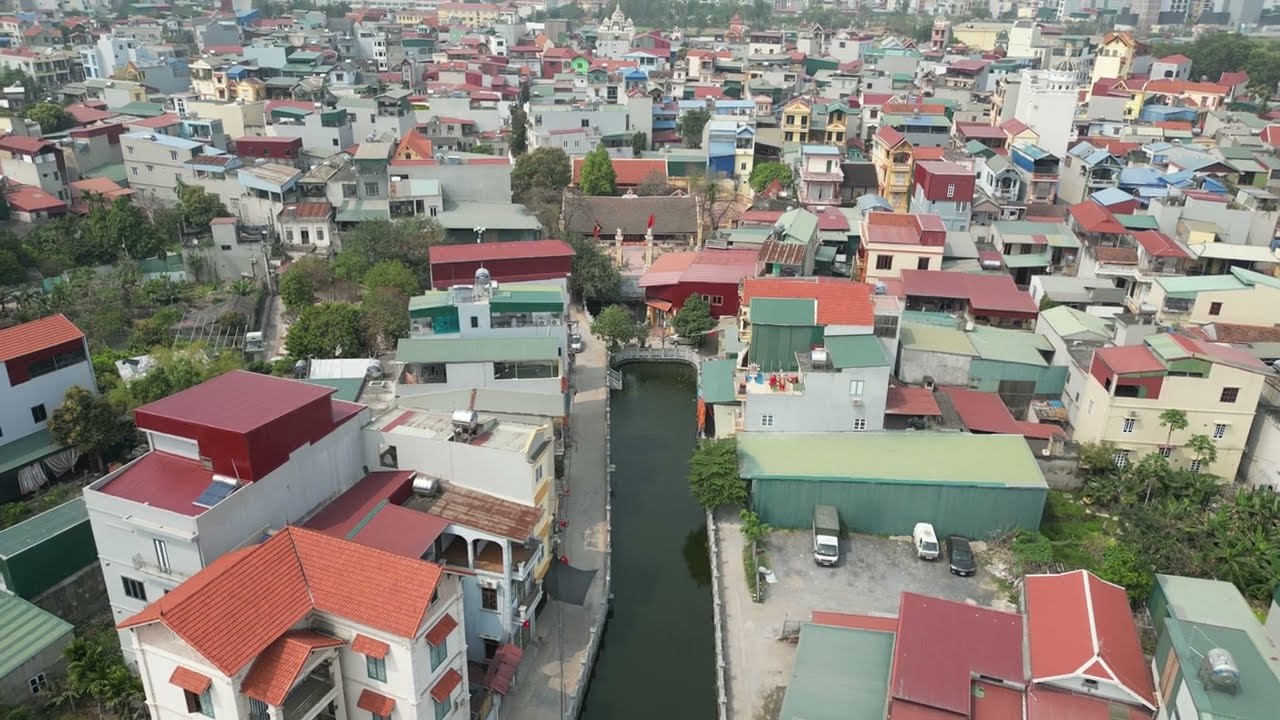The image is a photograph taken from a high aerial perspective, likely captured by a drone, depicting a crowded cityscape in what appears to be a foreign country, possibly Eastern Europe such as Poland or Ukraine. The city is characterized by a dense array of buildings that vary in height from one to four stories, with a mixture of green, red, orange, and white roofs. Many buildings also exhibit green facades, contributing to the vibrant, diverse color scheme. In the central part of the image, there is a notable waterway or canal flanked by these buildings, with a railing bordering the canal. The cityscape is dotted with parked cars and interspersed with trees, and there is a notable absence of major skyscrapers or modern glass buildings. Instead, the architecture appears traditional and somewhat foreign to Western eyes, including a temple with a domed roof. The photograph was taken during the daytime, with clear sunlight illuminating the entire scene.